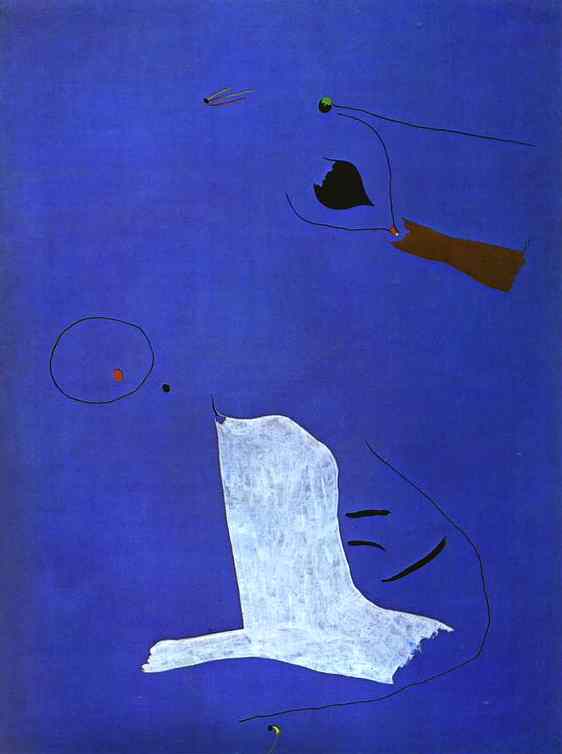This abstract piece of art, captured in a vertical photograph, features a vivid royal blue background. Dominating the bottom center of the painting is a large, white reverse T-shaped form, evoking images of a tree trunk or a primitive drawing of a sea otter. Surrounding this white shape, there are various black lines, including three distinct black strokes and a thin, backward-curving semicircle. 

To the left and slightly above the white figure, there is a red dot encircled by a thin black line, with an adjacent black dot outside the circle. The top right corner of the artwork contains a mix of additional shapes: a brown arm-like figure resembling a severed tree branch, a small black heart-shaped object, a green circle, and more delicate black lines intersecting in various directions. These elements add to the chaotic yet intriguing nature of the scene. 

The entire painting is infused with a playful and childlike energy, characterized by simple forms and vibrant colors, making it a captivating and whimsical abstract composition.